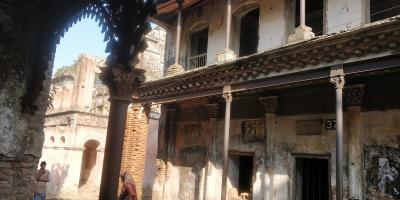The photograph depicts a weathered and possibly dilapidated two-story white stone building, which showcases its age through significant wear and muted shades of off-white, tans, and browns. The building features large openings for doors and windows both on the lower and upper floors, with no actual doors or window glass in sight. Thin metal or steel columns support the structure, particularly visible around the second-floor walkway.

To the left of the main building, a grand two-story archway stands prominently. Through this archway, another ancient and weathered building is visible in the distance, framed against a light blue sky. The scale of the archway is emphasized by the presence of a person standing within it, who appears to be about a quarter of the archway’s height. Another individual, possibly a woman wearing a head covering, can be seen from the side, approaching the archway.

Overall, the image seems to be captured with a low-quality device, adding a sense of timelessness and further highlighting the building's state of deterioration and the intricate yet worn architectural details.